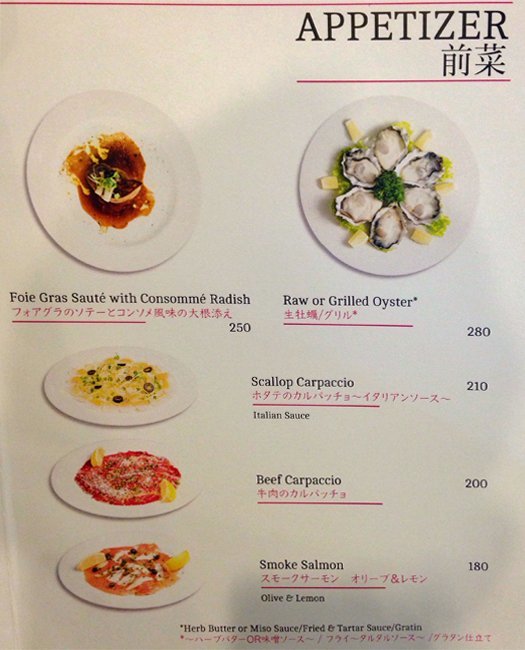This detailed image portrays the appetizer section of a fancier restaurant menu, featuring both English and possibly Asian script, likely Japanese or Chinese, with red text accompanying the descriptions. The menu showcases five exquisitely plated appetizer options. At the top left, there's Foie Gras Sautéed with Consomme Radish, and to the right, Raw or Grilled Oysters; both are depicted with overhead shots. Below these, three more dishes are illustrated from side views: Scallop Carpaccio, Beef Carpaccio, and Smoked Salmon. Each dish is labeled in English with the price ranging from $1.80 to $2.80. Additionally, there is a note indicating optional accompaniments such as herb butter, miso sauce, fried and tartar sauce, and gratin. The word "Appetizer" in bold black font is prominently displayed in the upper right corner, with corresponding Asian characters beneath it.